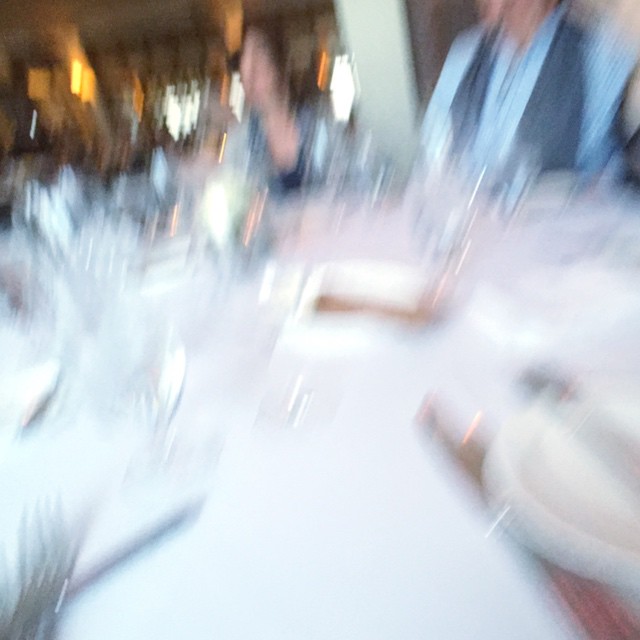In this image, taken inside a building, two individuals are seated at a bright white table. The blurry photograph captures what seems to be various glass objects scattered across the table. Both individuals are attired in blue – the man in a blue dress shirt accentuated by a blue vest, while the woman sports a blue shirt along with a light blue jacket. The background is a blend of dark yellowish-brown hues, highlighted by a white pillar positioned behind the pair. Through the window, the presence of sunlight suggests it might be morning or early afternoon. Despite the image’s blurriness, the dark yellow lights enhance the warm ambiance of the setting.